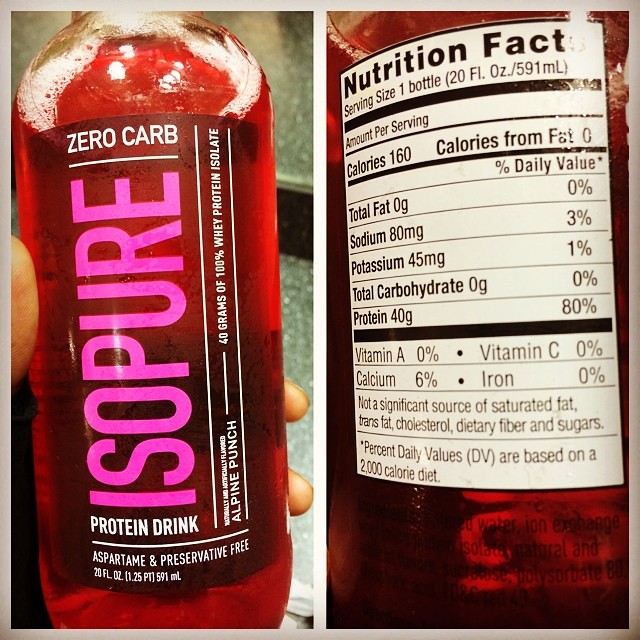**Detailed Descriptive Caption:**

The image consists of two panels showcasing a clear bottle filled with a red liquid, held by the light-skinned hand of a white person. The background is dark, enhancing the visibility of the bottle. 

In the left panel, the front of the bottle is displayed prominently. The label reads "Isopure" in pink letters at the top. Directly below in white letters, it says "Zero Carb Protein Drink." Additional information on the label includes "Aspartame and Preservative Free" and "20 FL OZ (591 mL) 1 PT 2.5 FL OZ," all written in white.

The right panel offers a closer view of the bottle's back, highlighting a white label adorned with black nutritional facts and other detailed information about the product. The label provides essential details and ensures transparency for those interested in the beverage's contents.